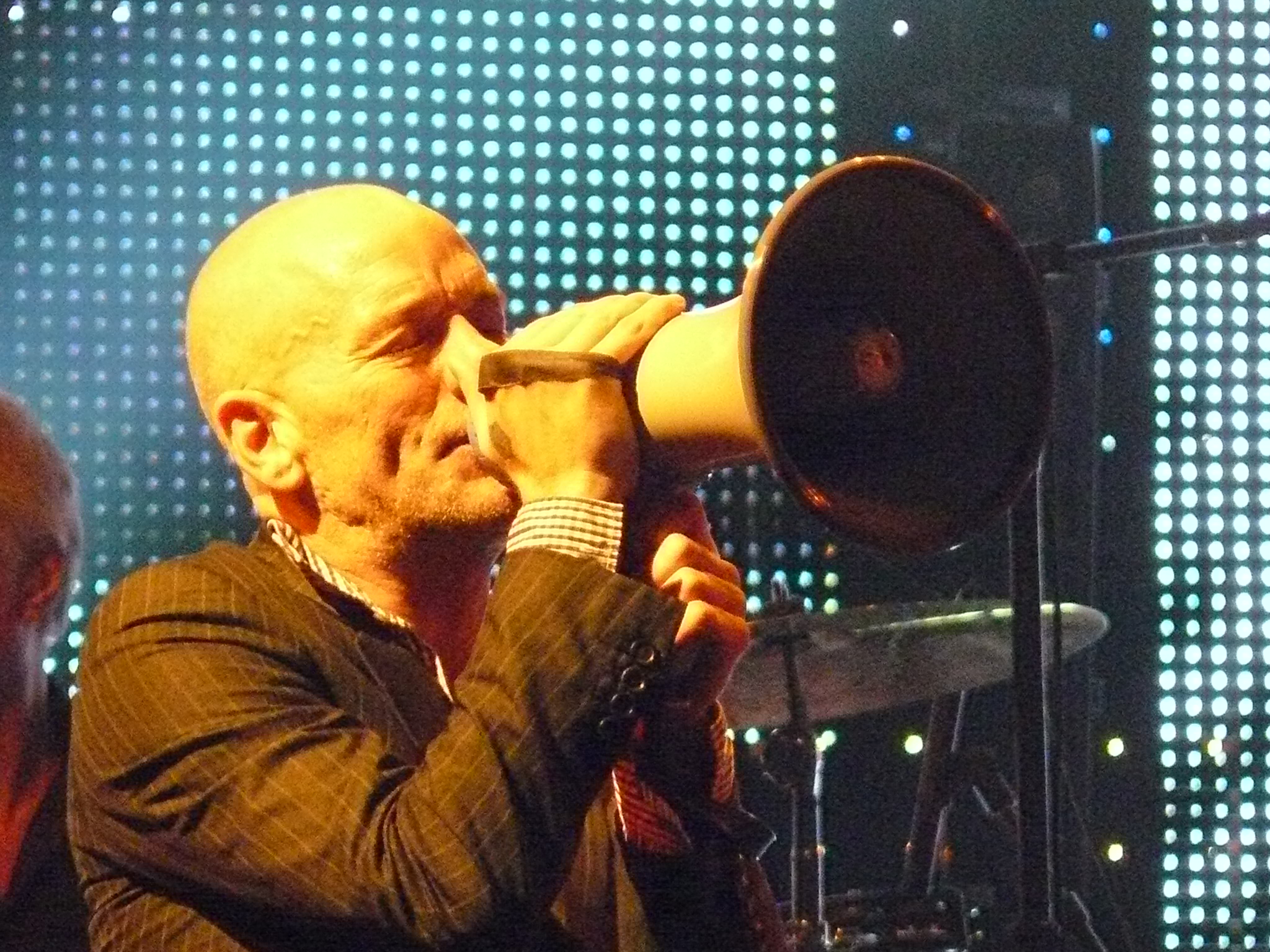This detailed photograph captures an older white male, reminiscent of the lead singer of R.E.M., intensely performing on stage. He is bald, with very light stubble and a prominent vein visible on the side of his head, highlighting his passion. He is dressed in a stylish black and white pinstripe suit jacket over a white and black striped collared button-down shirt. The man is holding a bullhorn, or megaphone, up to his mouth, seemingly singing or speaking into it. 

In the background to the left, another older male with gray hair and a black shirt can be partially seen, along with a drum set featuring a visible cymbal and microphone stand. The backdrop includes a wall adorned with digital lights in hues of white and blue, contributing to the vibrant stage ambiance. The image's colors span light blue, brown, silver, and a touch of orange, and it's challenging to ascertain if it was taken indoors or outdoors or during the day or night. The man, the primary focus, is facing towards the right, while the barely visible second individual appears to be facing to the left.